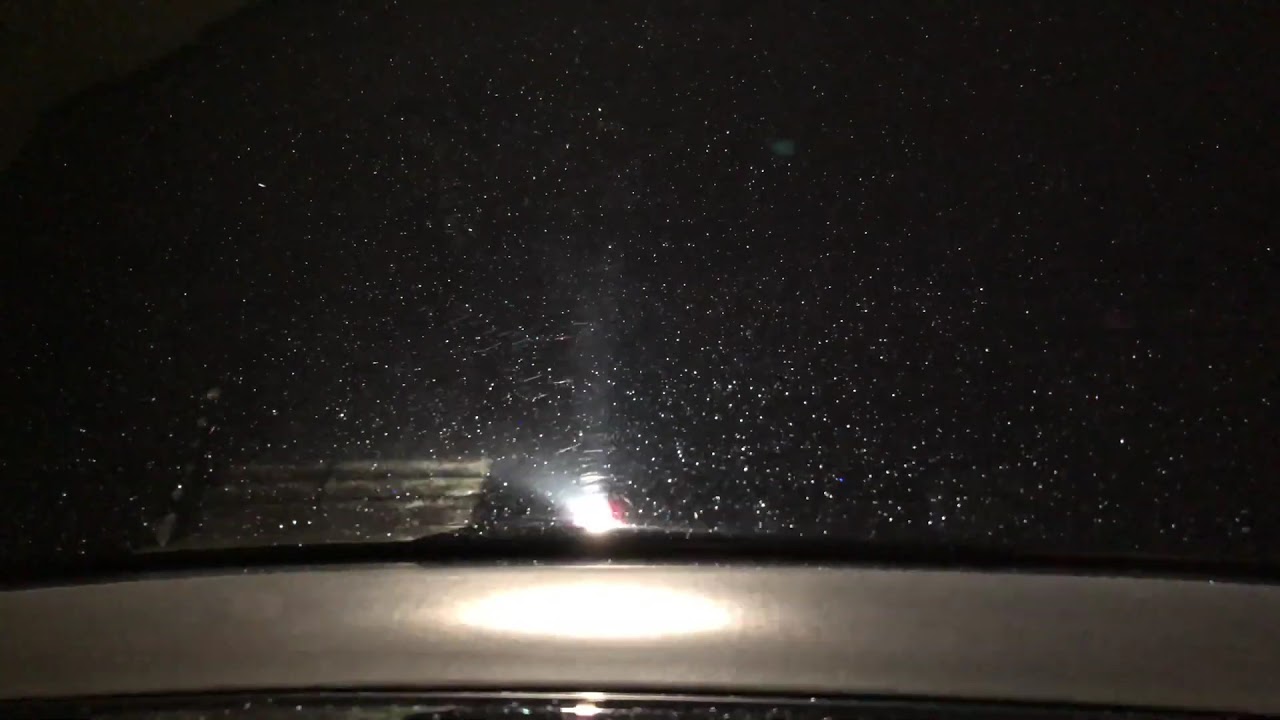The image appears to be challenging to interpret, likely taken at night, potentially from inside a car. In the bottom left corner, there's a metallic, slightly curved band that might be part of a windshield. Above this band, a light source is prominent, possibly from an oncoming motorcycle, due to it being singular. Surrounding the light, the image features a black area dotted with numerous white specks, suggestive of mist, water vapor, or a reflective surface rather than stars. Notably, to the left of the light source, a lighter region contrasts with the darker background, hinting at the reflection of the picture-taker's shadow. The overall scene lacks sufficient context, making it difficult to precisely identify the elements within.